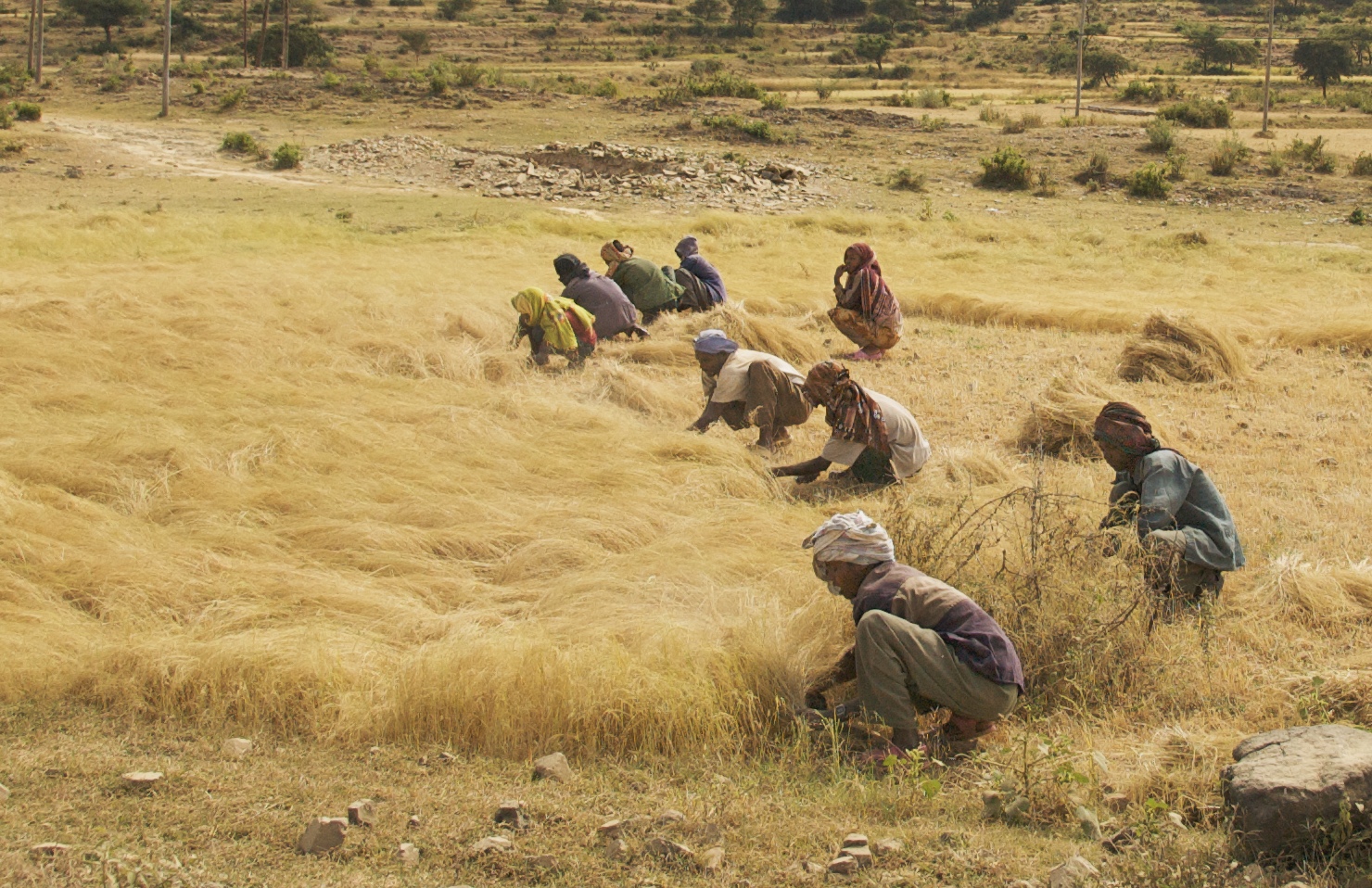The photo depicts a group of eight individuals, likely indigenous or African people, diligently harvesting a dry, wheat-like grass in a sun-scorched field. Positioned in a row stretching from the bottom to the top of the image, they are seen trimming and gathering the grass into neat piles on the ground. All workers sport head cloths, which seem to be worn to protect against the intense heat, and are dressed in variously colored shirts and cloths. The landscape is predominantly arid with patches of yellowed grass dominating the foreground, giving way to a dusty, desert-like setting with sparse green shrubs and barren trees in the background. A dirt trail winds through the scene, accompanied by an outcropping of rocks on the right side and partially visible tall structures, perhaps palm trees or power poles, emerging in the distant background.